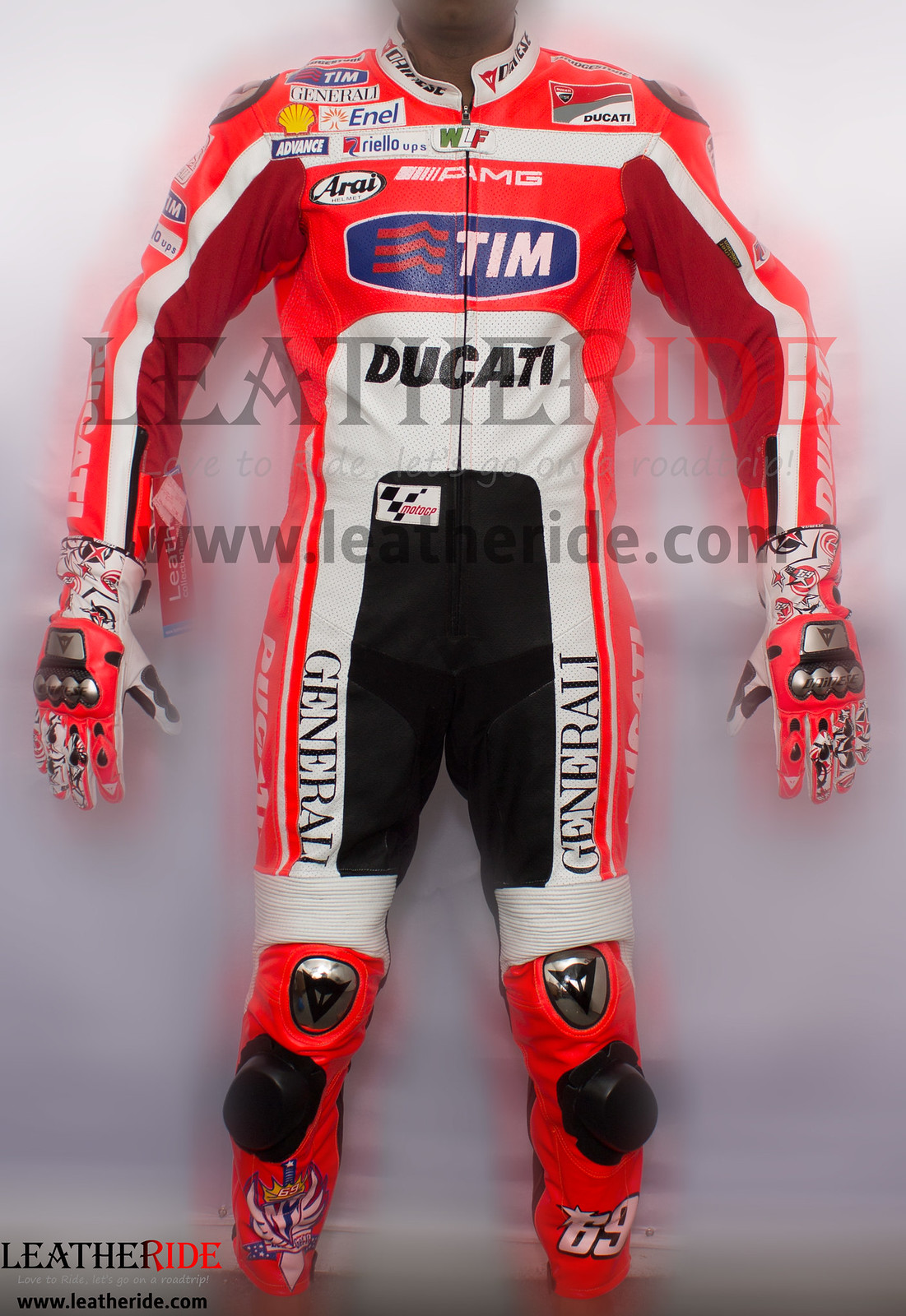This photograph captures a striking race car suit displayed on what appears to be a mannequin against a white wall. The suit is neon orangish-pink with prominent white stripes running down the arms, waist area, and knee regions. The inner crotch and leg areas are black, contrasting sharply with the rest of the ensemble. Across the chest, there's a blue oval patch with three red wavy stripes and the name "Tim" in white letters. The suit features multiple sponsor logos, including Ducati, Generali, Enel, AMG, Arai, and Leather Ride, with a mention of the website www.leatherride.com on the lower left side. It also incorporates practical details such as built-in metal knee and shin protectors, and reinforced gloves that match the suit's vibrant colors. The overall design is completed with a white collar, which adds to its visually dynamic appearance.